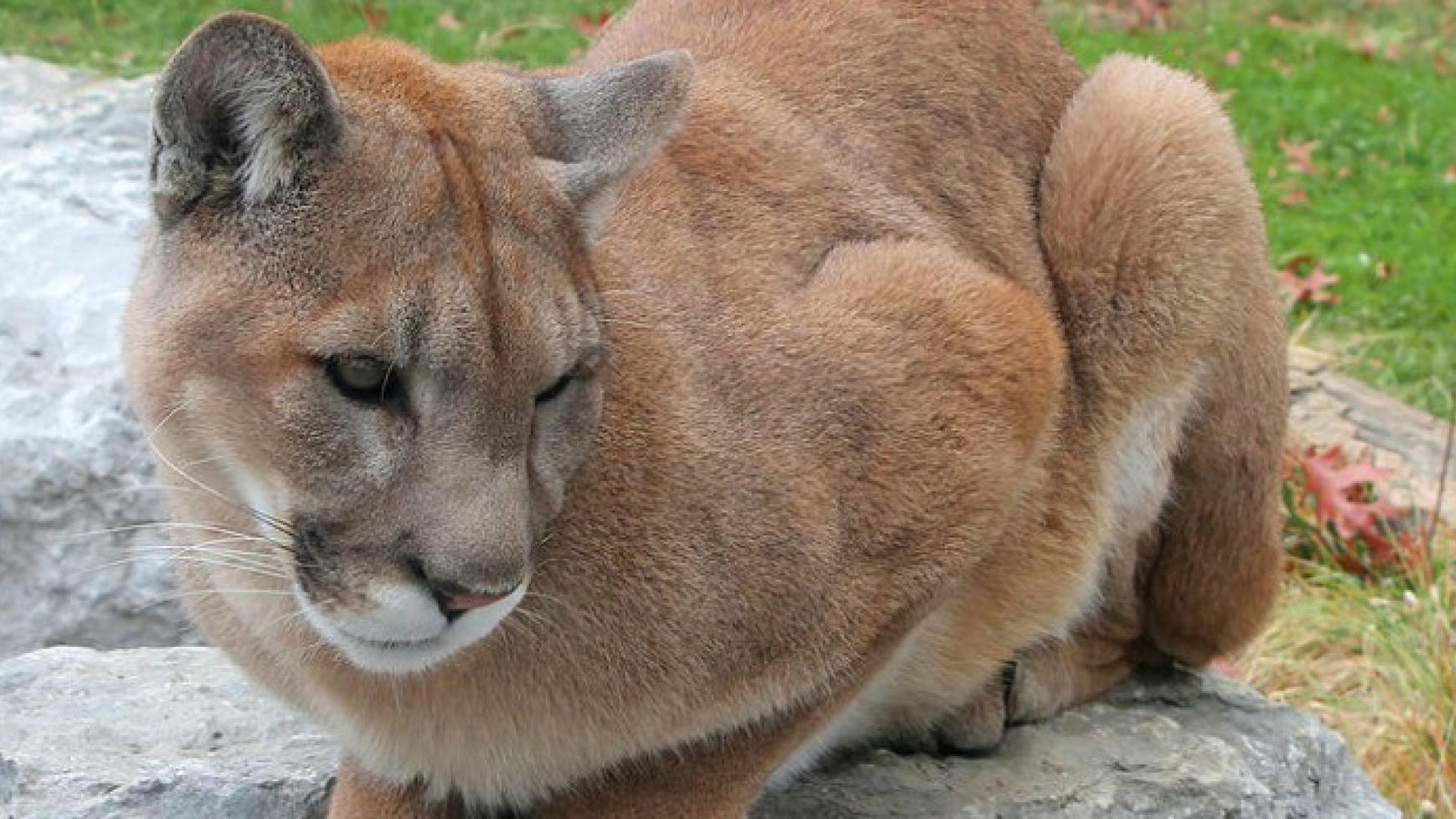This photograph features a beautiful, pensive female lion lying atop a gray rock. Her tan coat, accented with white fur around her muzzle and limbs, appears healthy and well-groomed. With her limbs tucked beneath her, she gazes thoughtfully off to her right into the distance, perhaps pondering her environment. The background comprises vivid green grass sprinkled with fall leaves, adding a touch of seasonal warmth to the scene. There might also be an artificial log, hinting that this might be a zoo enclosure. The close-up shot wonderfully captures the lion's regal and serene presence, filling most of the frame and highlighting her natural majesty in a clean and unique setting.